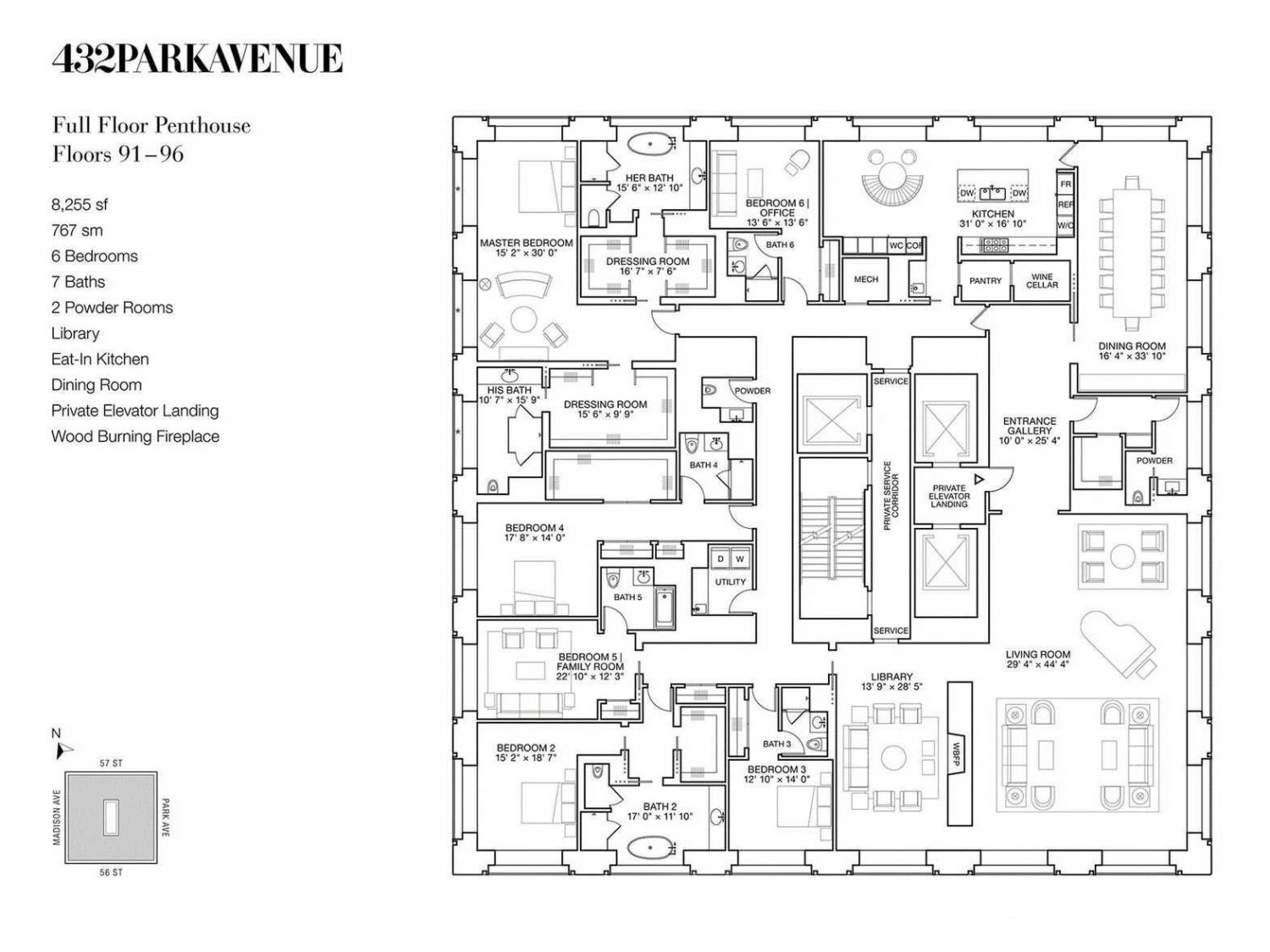This image is an overhead view of a detailed floor plan for a penthouse located at 432 Park Avenue. The penthouse spans floors 91 through 96 and boasts an impressive 8,225 square feet (approximately 607 square meters). The layout includes six bedrooms, seven baths, two powder rooms, a library, an eat-in kitchen, a dining room, and a grand living room that features a piano. Additional luxury amenities include a private elevator landing and a wood-burning fireplace. The diagram, labeled on the left-hand side and illustrated in black and white on the right, shows a comprehensive map of the sprawling space, highlighting its numerous rooms and the staircase that interconnects different levels. This penthouse epitomizes lavish living with a clear emphasis on spacious and well-defined areas for multiple functions.